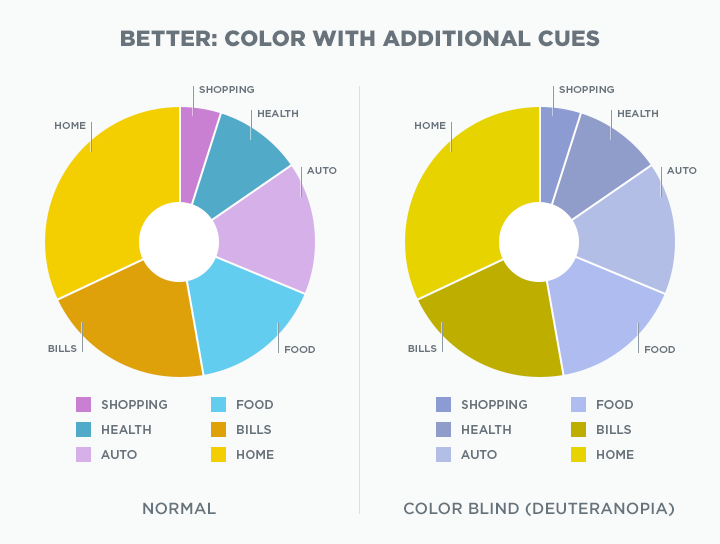The image features two side-by-side charts titled "Better Color with Additional Cues." On the left side, a pie chart illustrates categories such as shopping, health, auto, food, bills, and home, each section colored in distinct hues of pink, blue, and yellow. The chart on the right, labeled "colorblind (Deuteranopia)," shows the same categories, but the colors are muted and limited mainly to uniform shades of pea green, goldy yellow, and blue. This contrast highlights how individuals with normal vision perceive a variety of vibrant colors, while those with deuteranopia see a more monochromatic palette lacking in color variety. The left chart's largest section is 'home' in light yellow, followed by 'bills' in dark orange, 'food' in light blue, 'auto' in light purple, 'health' in dark blue, and 'shopping' in violet, showcasing detailed color cues understood from normal vision.